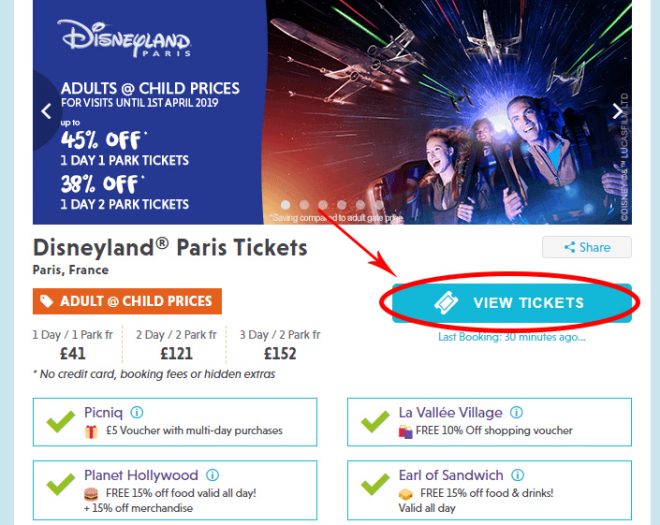An image from Disneyland Paris depicts a group of excited visitors strapped into seats on an exhilarating ride. Above them, futuristic spaceships can be seen soaring, emitting vibrant green and red laser beams. The entire scene is bathed in a blue hue on the left side of the image, emphasizing the dynamic and thrilling atmosphere of the adventure. 

Overlaying the image is a prominent promotional banner offering substantial discounts on Disneyland Paris tickets for visits until April 1st, 2019. It mentions up to 45% off on one-day, one-park tickets, and 38% off on one-day, two-park tickets. A light blue box labeled "View Tickets," circled in red with an arrow pointing at it, directs viewers to more ticket information.

On the left, additional text highlights specific ticket pricing: 
- One day, one park tickets for £41
- Two days, two parks tickets for £121
- Three days, two parks tickets for £152

The promotion also reassures potential buyers that there are no credit card booking fees or hidden extras, and includes a green checkmark indicating a £5 picnic voucher with multi-day purchases.